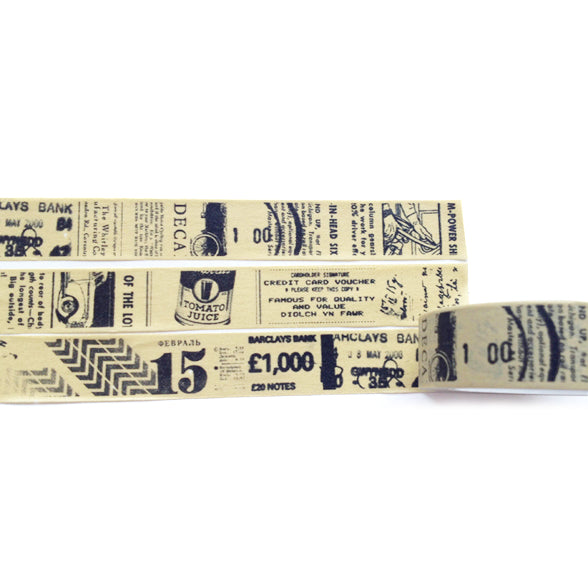The image showcases an assemblage of newspaper clippings, appearing to be long strips of roughly cut paper with a vintage aesthetic, featuring a mix of labels and text. The paper has a yellowy tint, suggesting age, and the printing is somewhat rough. Each strip contains black text and various images on a grayish-white background. Prominent among the text are multiple mentions of "Barclays Bank" and references to monetary values in Euros, such as "European 1000" and "European 20 notes." One strip prominently features a central piece reading "DECA 100." This strip also includes an image of a can labeled "tomato juice" with bold black text inside a white-bordered frame and some tire tracks paired with the number 15 next to a "1000€" symbol. The clippings appear to have a somewhat disjointed arrangement with three strips aligned orderly and one protruding at the bottom right, suggesting they might be attached to a surface, possibly decorative scotch tape. Some strips also bear banking stamps and circular rings, adding to the sense of their origin and use.